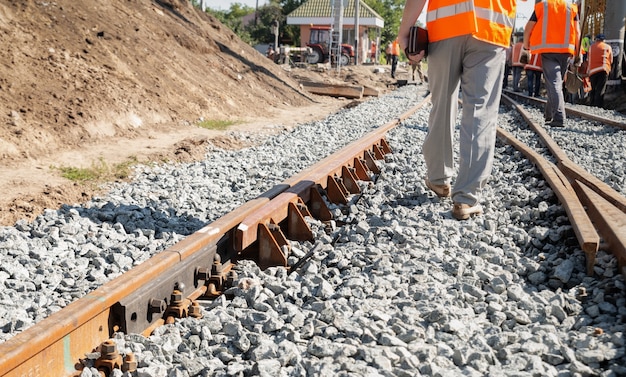The image depicts a ground-level view of train tracks lined with light-colored gravel. In the foreground, a man in gray pants and an orange safety vest walks along the tracks, holding a black object. The tracks, surrounded by large gravel, diverge to the right, with metal bars visible. To the left of the tracks is a mound of dirt that inclines upward. In the upper right background, several city or train workers, also in orange vests, huddle together in conversation. Farther back, near the left-center of the image, stands a small building with a white roof and red siding, possibly a station or utility hut, with a tractor parked in front of it. The scene is bustling with activity amid the construction or maintenance work being carried out on the railway.